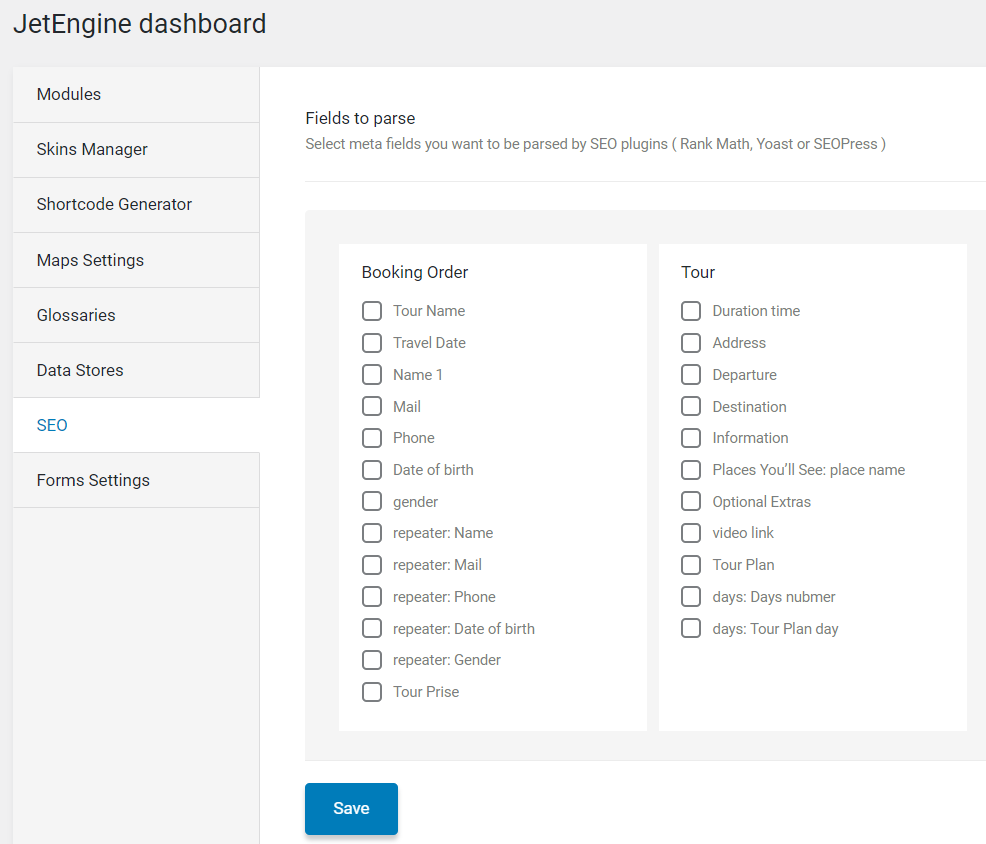In this screenshot, the JetEngine Dashboard is displayed prominently at the top in black text, contrasting against a predominantly grey and white backdrop. The interface design includes a blue 'Save' button located towards the left side of the screen, with another identical 'Save' button placed towards the center for easy access.

Below the JetEngine Dashboard title on the left-hand side, there is a navigational list comprised of several items in sequence: Modules, Skins Manager, Shortcode Generator, Maps, Settings, Glossaries, Data Stores, followed by a blue-highlighted item labeled 'SEO' within a white box background. Continuing below in the same list in grey again are Forms and Settings in black text.

To the right of this navigation menu, the screen primarily features a large white section titled "Fields to Parse," written in black text. Directly under this heading, it prompts the user to "Select Metafields you want to be parsed by SEO Plugins," listing options such as Rank Math, Yoast, or SEO Press. 

The main content area is divided into two columns. The left column lists a series of metafields under "Booking Order," including:
- Tour Name
- Travel Date
- Name 1
- Mail
- Phone
- Date of Birth
- Gender
- Repeater: Name
- Repeater: Mail
- Repeater: Phone
- Repeater: Date of Birth
- Repeater: Gender
- Tour Price

The right column is titled "Tour" and contains similar categorized options, each accompanied by selection boxes. These options include:
- Duration
- Time
- Address
- Departure
- Destination
- Information
- Places You'll See
- Place Name
- Optional Extras
- Video Link
- Tour Plan
- Days
- Days Sub Number
- Days Tour Plan Day

This detailed layout ensures that users can efficiently navigate through the various settings and options available within the JetEngine Dashboard for customizing and managing their content.